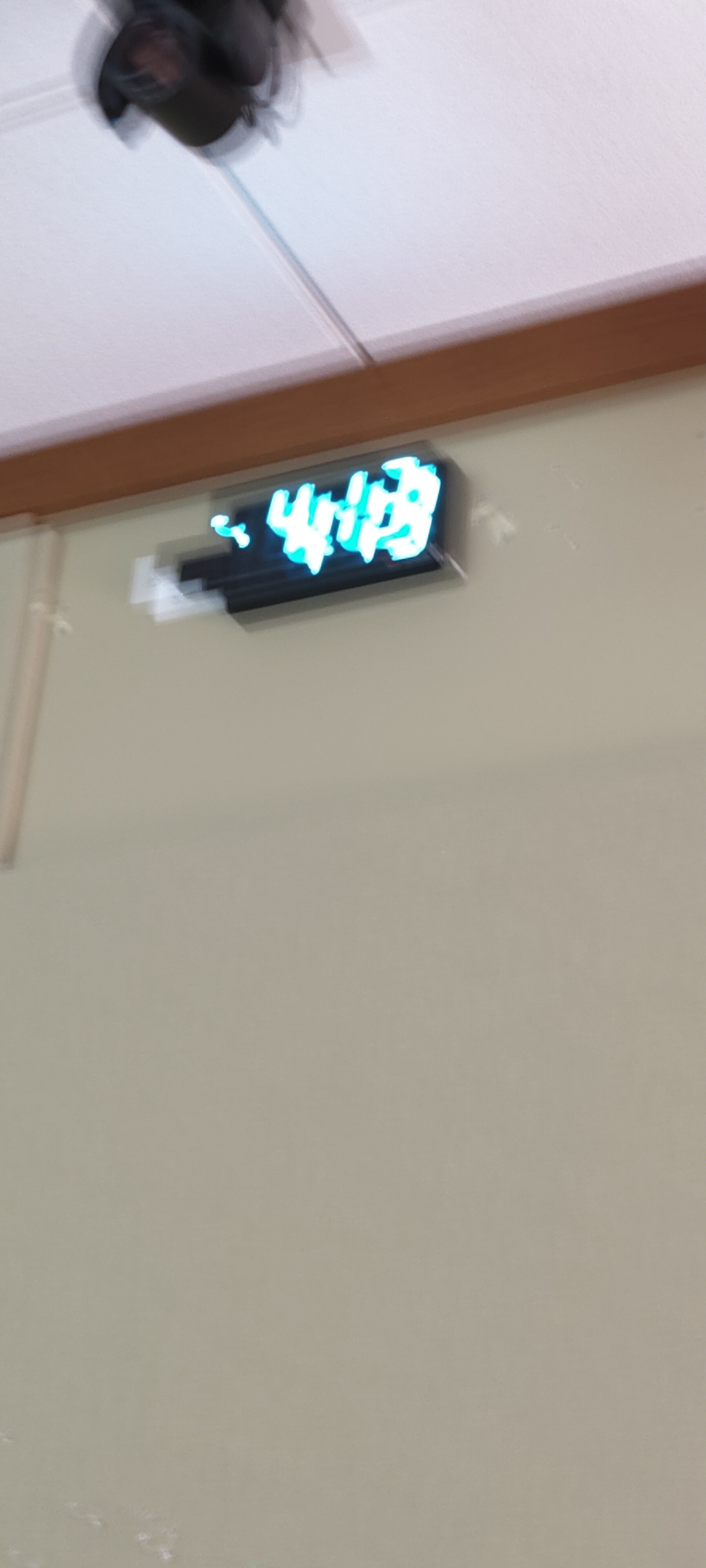This is a blurred cell phone photograph with a long aspect ratio, capturing a digital clock mounted very high on a beige wall, almost where the wall meets the white-tiled ceiling. The clock displays the time as 4.13 in large, luminescent blue digits, though the image is doubled due to motion blur. Along the upper edge of the wall, a wooden molding separates it from the ceiling. In the top left corner of the image, there appears to be a small black light fixture, possibly connected to a nearby outlet. The overall composition suggests a high-angle point of view, with additional details like a black string or cord possibly leading to the clock, enhancing the complexity yet maintaining the primary focus on the digital clock and its distorted display.